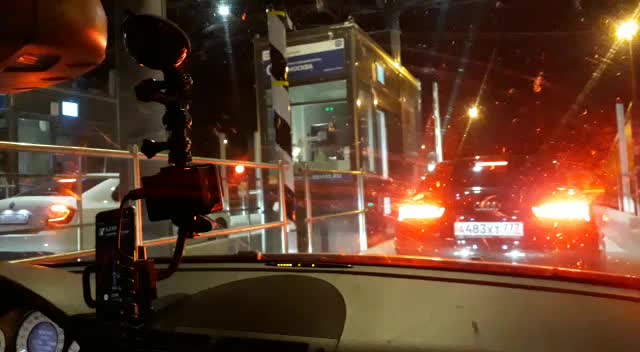A night-time image captured from inside a car, possibly using a dash cam, shows an interior view featuring parts of the dashboard, including gauges visible on the left and an unidentifiable contraption in the center, likely a phone holder or camera. The main scene beyond the windshield depicts the situation at a toll booth. Directly ahead, a darker car, with its brake lights engaged, is positioned in front of a silver toll booth adorned with an unreadable blue and white sign. To the left, another white car, also at a toll booth with its brake lights on, can be seen. Both toll booths are flanked by white and black striped poles and metal railings. The entire scene is illuminated by streetlights, against a backdrop of a dark, night sky. The license plate of the darker car reads 483X.